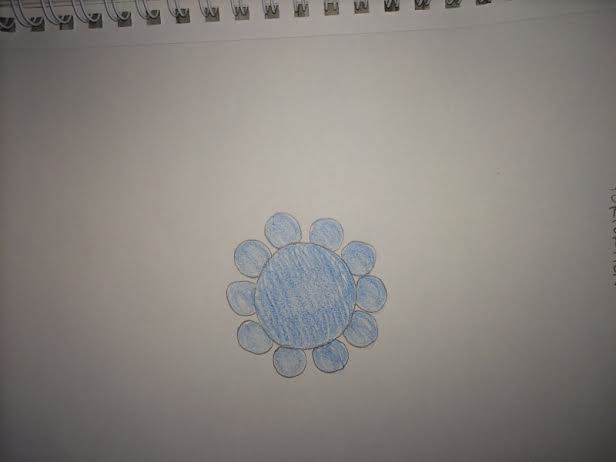The photograph captures a hand-drawn illustration on an off-white, creamish sheet of paper, attached to a horizontally placed spiral-bound notebook. The top edge of the image reveals the silver metal of the spiral binding along with the corresponding square cutouts of the pad. Central to the image is a simplistic drawing of a flower, sketched within a space starting approximately 15% from the bottom and extending up to about 50% of the height of the paper. The flower consists of a large, circle at the core, completely shaded in medium blue, with a subtly darker, wobbly outline suggesting added detail or a previous drawing attempt. This central circle is surrounded by ten smaller, equally spaced blue-shaded circles, forming the petals. The strokes used in the sketch are mostly vertical, possibly drawn with a crayon or colored pencil. The overall image is of low resolution, appearing slightly grainy and pixelated, which affects the true color representation. The background is plain, with no text or additional markings, and the photograph is dimly lit, hinting at an indoor setting.